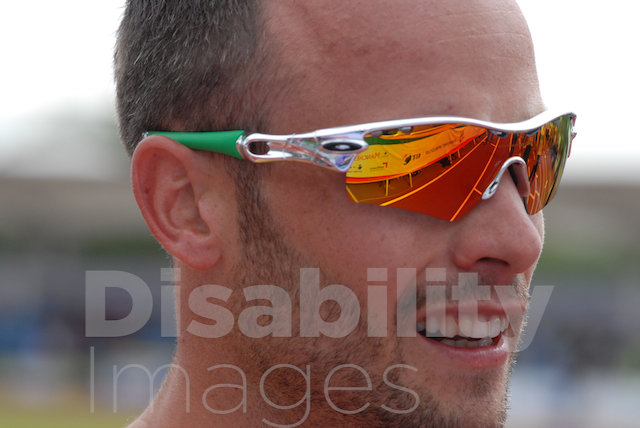The close-up photograph features a Caucasian man, likely in his mid-30s, with closely cropped brown hair that contains flecks of white and gray, and a short, neatly trimmed beard and mustache. His skin is tanned, indicating time spent outdoors. The man is sporting a unique pair of Oakley sunglasses with silver frames and bright green silicone tips behind the ears. The lenses are a reflective wraparound style with a striking yellow-to-orange gradient. Reflected in the mirrored lenses is a racetrack and some banners, suggesting he might be at an athletic event. His expression appears to be one of concentration or confusion, likely captured mid-speech. The background of the image is blurred, obscuring any additional context. Superimposed over the photo are the words "disability images," in bold and non-bold text, respectively. The focus is solely on his head and face, providing no further context about any disabilities he may have.